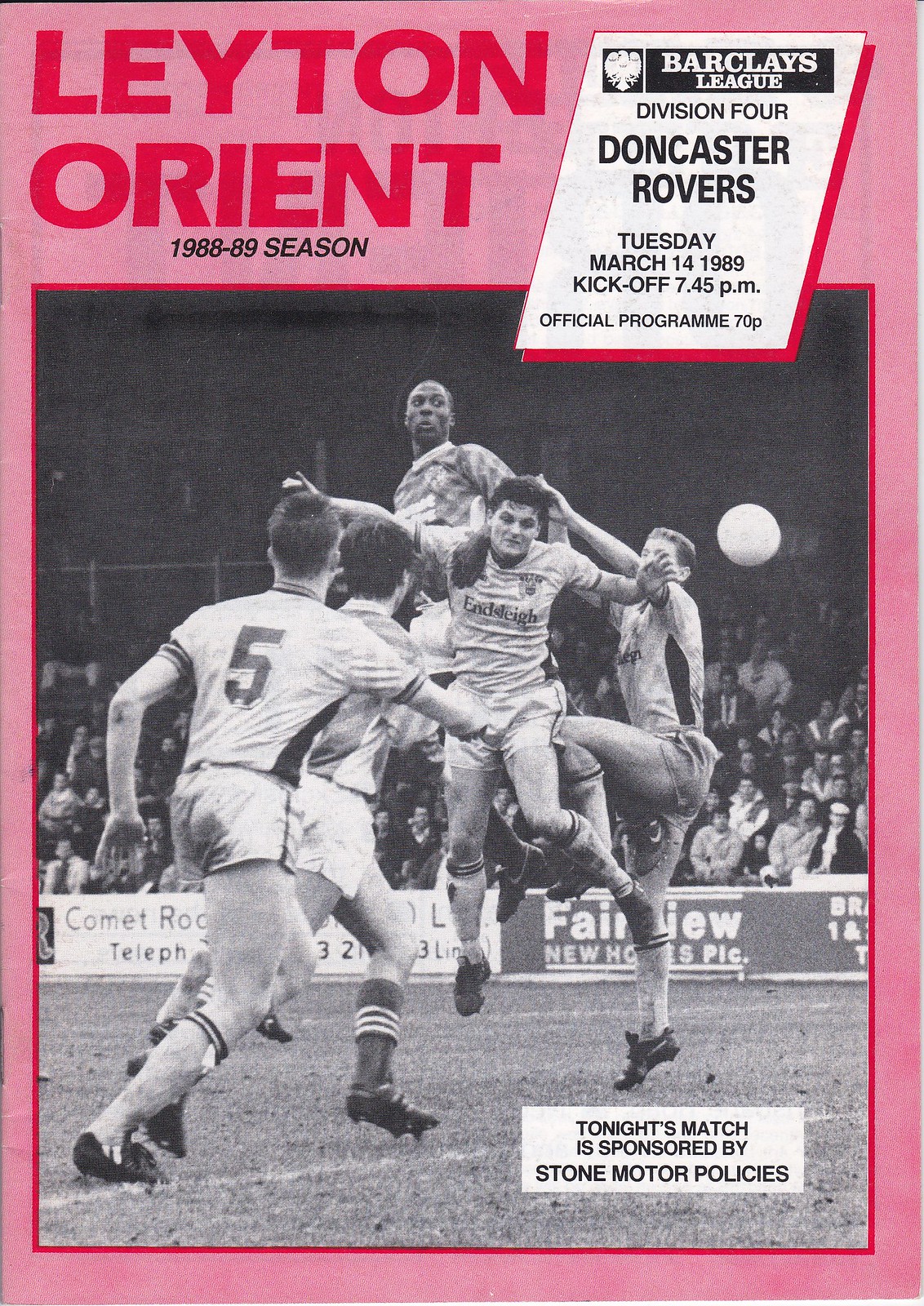This striking cover of Leighton Orient's soccer club program for the 1988-89 season presents a vivid, black-and-white outdoor photograph capturing the intensity of a live match. The image, set against a bold pink background, shows a group of dirty, soil-covered players fiercely contending for the ball, which hovers in the air just above their shoulders. The chaotic scene features one player kneeing another in the upper thigh and an elevated player seemingly defying gravity, demonstrating the high stakes and physicality of the game. Enthusiastic fans, some on their feet, fill the background, along with visible advertising banners for Fairview and Comet. Text details on the cover announce the upcoming Barclays League Division 4 match between Leighton Orient and Doncaster Rovers, scheduled for Tuesday, March 14, 1989, with a kickoff at 7:45 pm. An official program notation, priced at 70 pence, appears alongside the message “Tonight's Match is sponsored by Stone Motor Policies,” completing this evocative and historical depiction of British football.